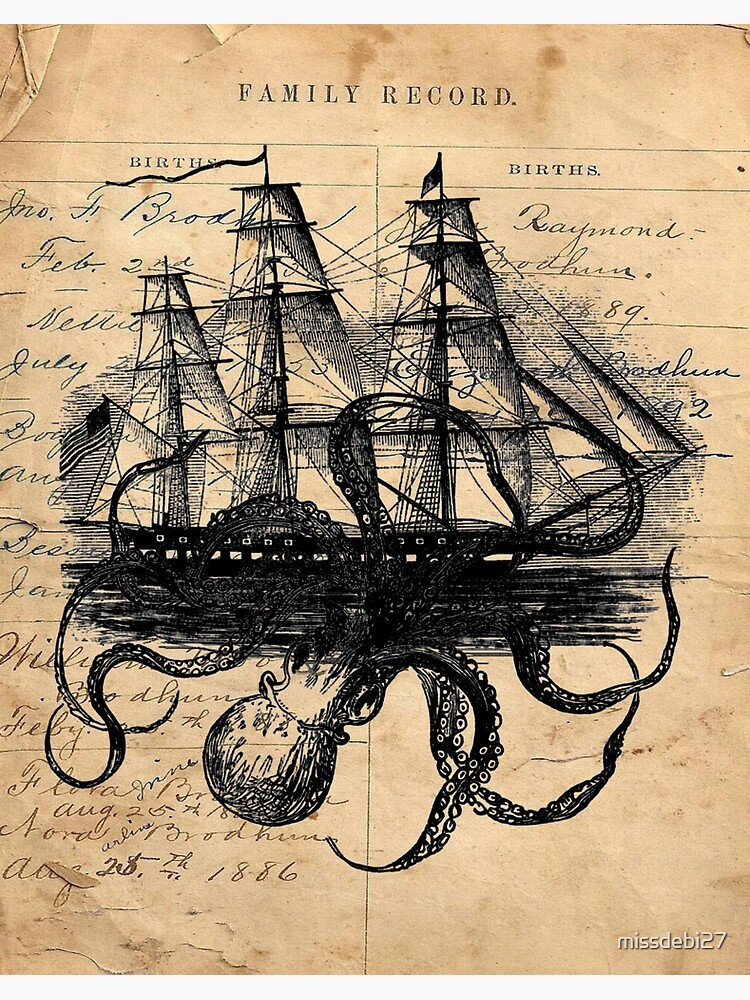This image depicts a vintage-styled, yellowed, and worn piece of paper, appearing to be from the mid-1800s, labeled at the top in black lettering as "Family Record." It features two columns titled "Births" in elegant calligraphy, though much of the names and dates, such as a visible entry of "August 28, 1886," are obscured by an intricate, hand-drawn pen and ink illustration. The artwork showcases a three-masted schooner with fully deployed sails and an American flag flying at the stern. The schooner is dramatically ensnared by a gigantic, upside-down octopus, whose lengthy tentacles envelop the ship on all sides. The ship and sea creature are rendered in black and white, adding to the antique feel of the image. The bottom right corner features the inscription "Miss Debbie 27," likely indicating the artist or uploader of the document.